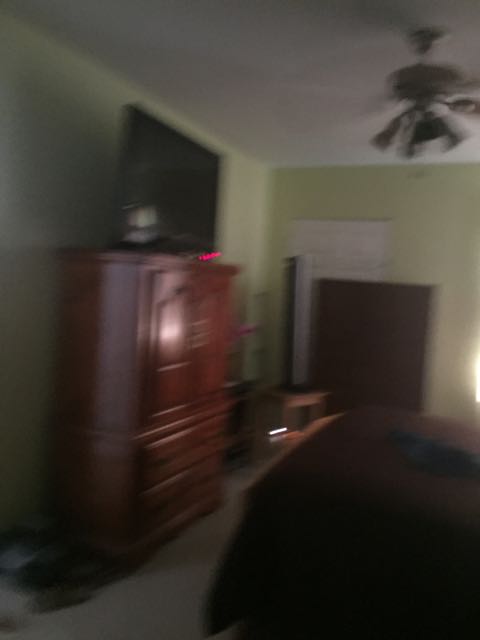This image captures a very out-of-focus, blurry photograph of an interior bedroom. The room has light green walls and a white ceiling. A dark shape in the lower right-hand corner appears to be a full-size bed with a light wood frame and a dark bedspread. Above the bed, a ceiling fan is visible. 

Along the back wall, there seem to be a white doorway and a wooden dresser with two bottom drawers and cabinet doors above, topped with a miscellany of objects including a thin, bright rosy red streak. A flat-screen TV, nearly touching the ceiling, is high on the left wall, mounted atop the aforementioned dresser or armoire. Additionally, there seems to be a table with what looks like a dehumidifier and some shoes scattered below. The flooring appears to be gray carpet.

In the distance, possibly near the corner of the room, there is an object that could be a fireplace or a picture on the wall, and below it, a book cabinet. The overall illumination of the room is faint, with a possible white table light providing some brightness in the right corner.